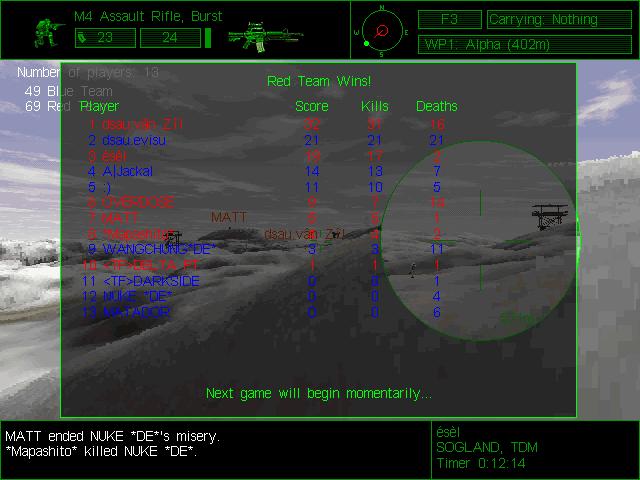This screenshot from a military-themed video game captures the victorious moment for the Red Team. Superimposed over a rough, snowy landscape with hills and grassy knolls, a semi-transparent dark black window displays detailed game statistics. At the top of this overlay, bold green text announces "Red Team Wins," beneath which appears a ranked list of players, each accompanied by their scores, kills, and deaths highlighted in green. A smaller, lighter gray circle within this rectangle seems to magnify a part of the background, revealing a tower and a white structure or aircraft. The screen's top and bottom margins are framed in black bars. The upper bar includes green text displaying game stats such as a soldier's status, a compass, and a weapon icon labeled "M4 Assault Rifle Burst" with counts "23 and 24". The bottom bar provides live updates such as "Matt Ended Nuke DE’s Misery" and other player actions. Across the bottom center, green text alerts players that "Next Game Will Begin Momentarily."